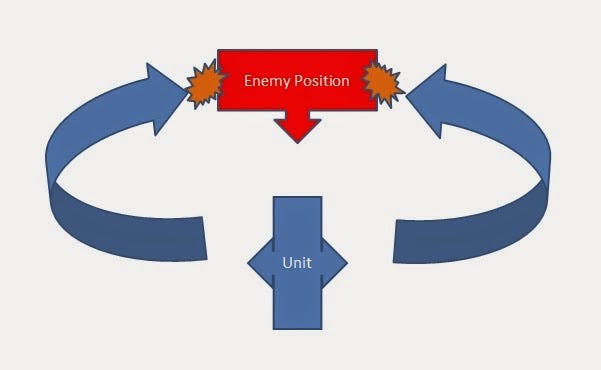The image depicts a simple, rectangular diagram with a white background. At the top center, there is a red rectangular box labeled "enemy position" in white text. Emerging from the bottom of this red box is a downward-pointing arrow. Flanking this red box on both sides are orange spiky blobs, reminiscent of comic book "BAM" symbols, with blue jagged outlines.

From the left and right sides of the diagram, two blue curved arrows extend upwards and converge towards the red "enemy position" box. These arrows are light and dark blue and have flat bottoms. At the bottom center of the diagram is an inverted blue rectangle, labeled "unit" in white text, featuring arrow-like fins on either side. The overall structure emphasizes a clear interaction between the unit at the bottom and the enemy position at the top, with the arrows indicating movement and engagement direction.